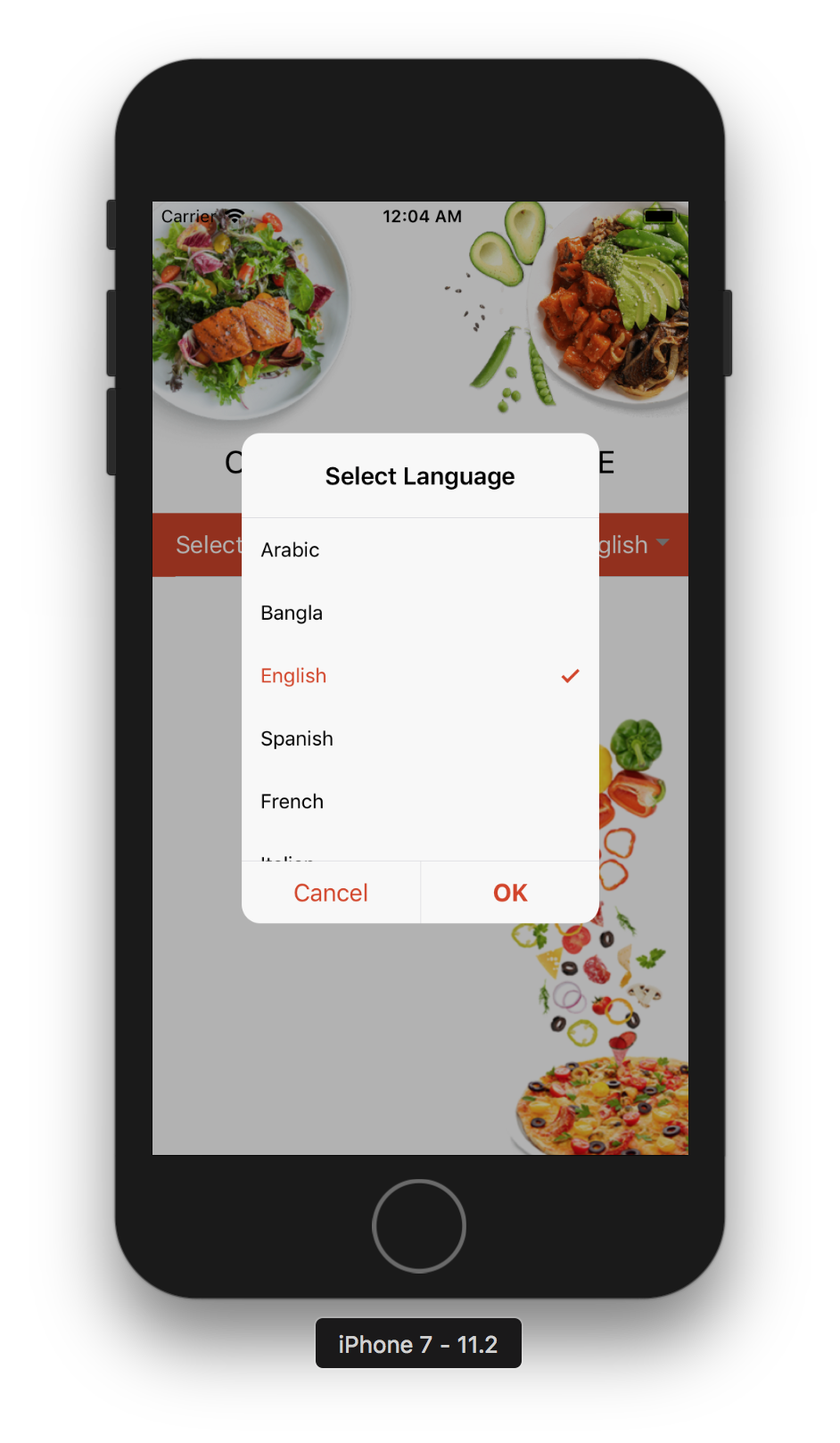The image displays a black iPhone 7, with the time reading 12:04 AM. The screen shows a food delivery app that features a menu bar at the center, prompting the user to select a language from options including Arabic, Bangla, English, Spanish, and French. The user has chosen English, highlighted in red with a check mark. 

At the top of the screen, a white plate adorned with a fresh vegetable salad and a piece of salmon cut into two portions is visible. Below this, another plate features a colorful assortment of fruits and vegetables, including kiwis, avocados, carrots, and peas. Further down, various illustrations of vegetables like tomatoes, broccoli, onions, and cheese are present. 

At the bottom right corner of the phone's screen, an appetizing pizza topped with black olives, red onions, green onions, cheese, and possibly banana peppers is showcased, tempting the senses with its savory ingredients.